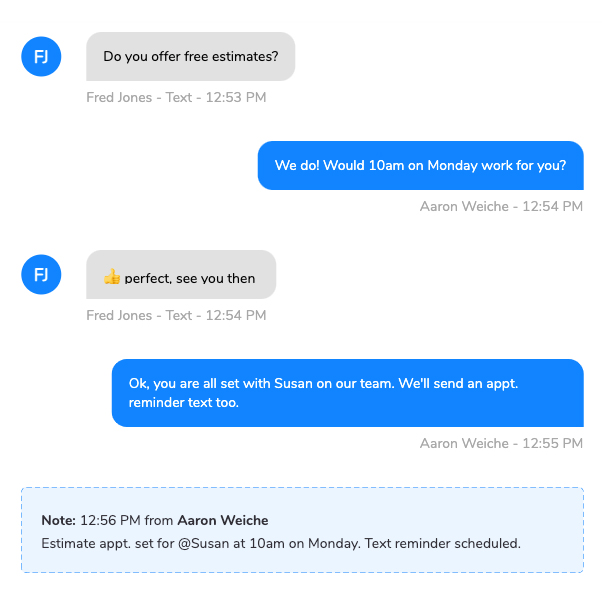A screenshot of a text message conversation shows an exchange between Fred Jones and Aaron Weish. The conversation initiates with Fred Jones' message at 12:43 PM and 12:53 PM, asking if free estimates are offered. At 12:54 PM, Aaron Weish responds affirmatively and proposes a meeting at 10 AM on Monday. Fred Jones replies with a thumbs-up emoji and texts "Perfect, see you then." Fred’s messages are displayed in light blue with a gray background, while Aaron's responses have a blue background with white text. At 12:55 PM, Aaron confirms the appointment, stating, "You're all set with Susan on our team. We'll send an appointment reminder text, too." This is followed by an informational note at 12:56 PM from Aaron, confirming the estimate appointment set with Susan at 10 AM on Monday and noting that a text reminder is scheduled. The conversation ends with this final piece of information.